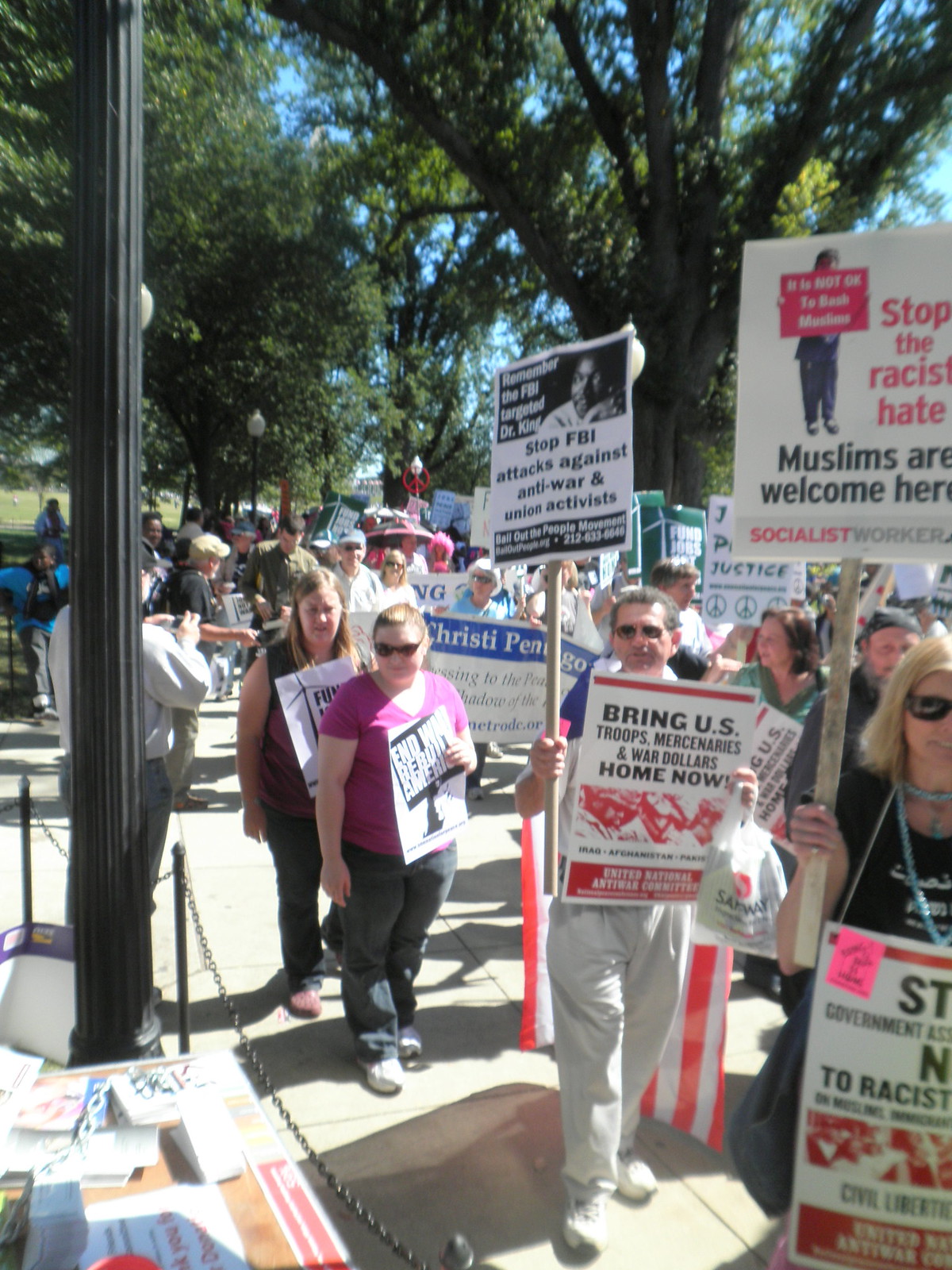The photo captures a peaceful protest occurring in a picturesque, sunny park with lush greenery and an open field in the background. The scene is quite crowded with likely dozens, if not hundreds, of participants, consisting primarily of men and women, many appearing to be suburban liberals based on the demographic noted. Protesters are holding a variety of signs, some on poles and others across their chests. Prominent messages include "Stop FBI attacks against anti-war and union activists," "Bring U.S. troops, mercenaries, and war dollars home now," "Stop the racist hate. Muslims are welcome here," and a reference to the Socialist Workers Party. A black lamppost stands on the far left, and an information table with literature is visible, set behind a chain-link partition. The demonstration likely focuses on themes of anti-war, social justice, and anti-racism, reminiscent of the activism following the 9-11 attacks. Most protesters are dressed for a sunny day, many wearing sunglasses, and the atmosphere is charged with a call for peace and justice.